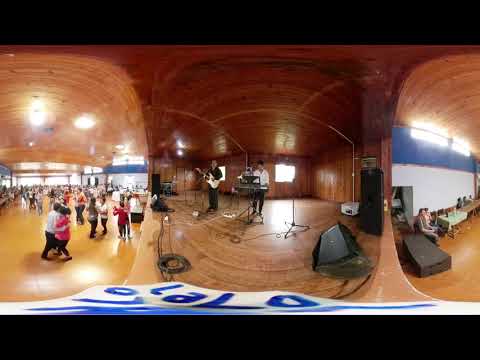The image depicts a cavernous dance hall or gymnasium with a distinct wooden aesthetic, featuring wooden floors, walls, and ceiling. The photo appears to be a 360-degree VR capture that includes some black rectangular framing at the top and bottom. On the left side, a crowd of people, including a couple in white and red who are hugging and dancing, suggests an ongoing dance or ceremony. Several other couples are also dancing nearby. The center of the room is occupied by a band, with a bass player and a keyboard player on a wooden stage. There is a microphone setup indicating a live performance. To the right side of the image, a few people are seated, possibly near a refreshment table or waiting area. The entire scene is bustling with activity, with many people milling about, especially behind the dancing couples.